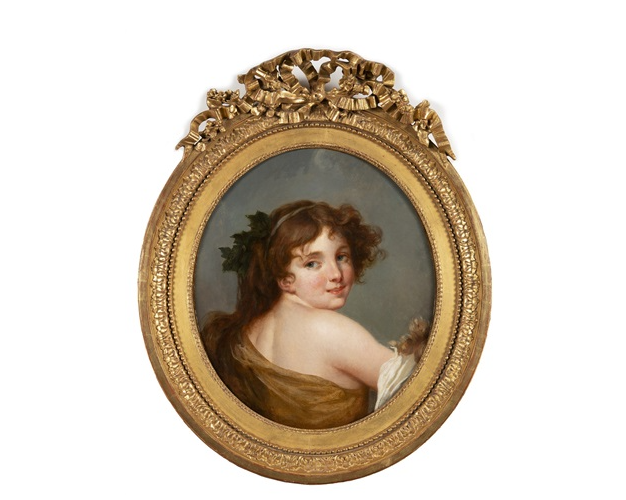The image features an intricate, golden, oval-shaped frame adorned with floral patterns on the top and delicate edging of small dots along the sides. Inside the frame is a detailed portrait of a young woman with dark brown, wavy hair styled with a leafy, holly-like trellis headband. She is depicted with her back partially turned, looking over her bare right shoulder toward the viewer. The woman is dressed in a brown-beige gown that leaves one shoulder exposed, with a white sleeve visible over her right elbow, above which golden-colored flowers can be seen. The background of the portrait is a dark green, which contrasts with the rich colors of her attire and the ornate frame.